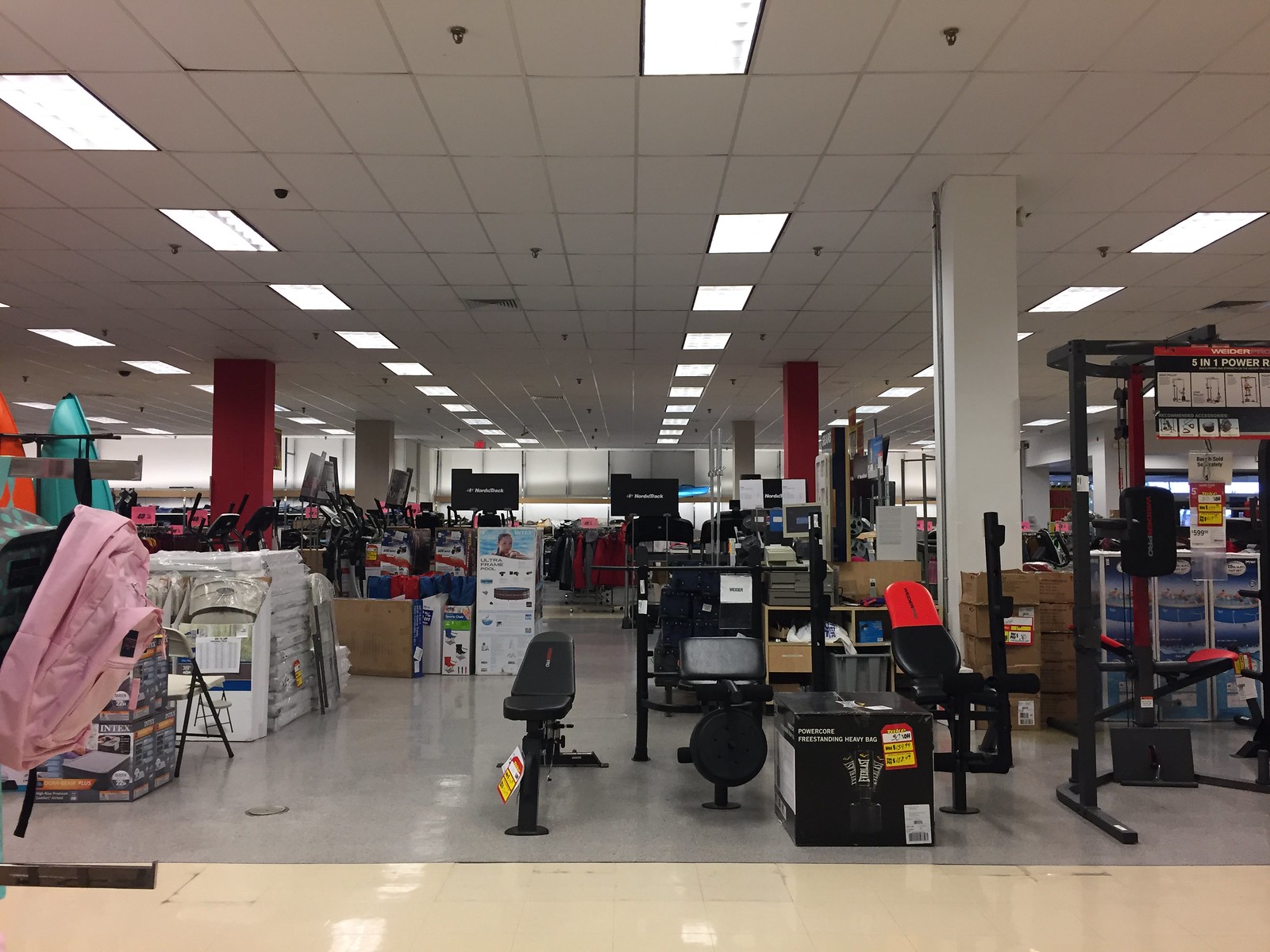This image showcases the interior of an expansive department store, resembling a Marshalls, Ross, or Burlington Coat Factory, featuring a diverse selection of goods. The spacious area prominently displays an array of gym equipment in the foreground, including weightlifting benches, black-framed square tube weight machines, and multifunctional fitness stations. On the left side, there's camping gear such as backpacks—with a distinct pink one standing out—alongside white folded chairs and various other outdoor items. To the far right, two kayaks—one blue and one orange—are propped against the wall. The store is characterized by white ceiling panels adorned with rectangular fluorescent lights aligned in a grid pattern, interspersed with red and white support pillars. Toward the back, there is a white-boxed swimming pool and stacks of mattresses. Completing the scene, the back wall features black posters and multiple racks of clothes, emphasizing the store's wide-ranging inventory of sporting, recreational, and home goods.